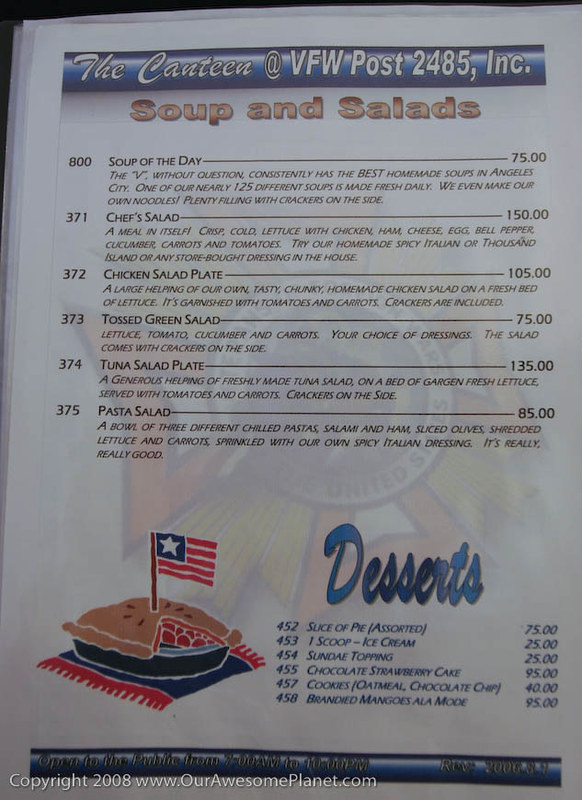Close-up of an indoor color photograph capturing a detailed view of a restaurant menu. The top section of the menu features a blue rectangular banner with white lettering that reads "The Cantina at VFW Post 2485, Inc." Below this banner, there is a section titled "Soup and Salads" in red lettering, followed by a list of menu items:

1. Soup of the Day priced at $5.57, item number 800.
2. Chef Salad priced at $1.50, item number 371.
3. Chicken Salad Plate priced at $1.05, item number 372.
4. Toasted Green Salad priced at $0.75, item number 373.
5. Tuna Salad Plate priced at $1.35, item number 374.
6. Pasta Salad priced at $0.85, item number 375.

In the lower right corner, there is a simplified drawing of an apple pie with a small American flag sticking out of it. To the right of the drawing, "Desserts" is written in blue script, followed by a list of six dessert items. An overlay print in the lower left corner reads "Copyright 2008 www.ourawesomeplanet.com."